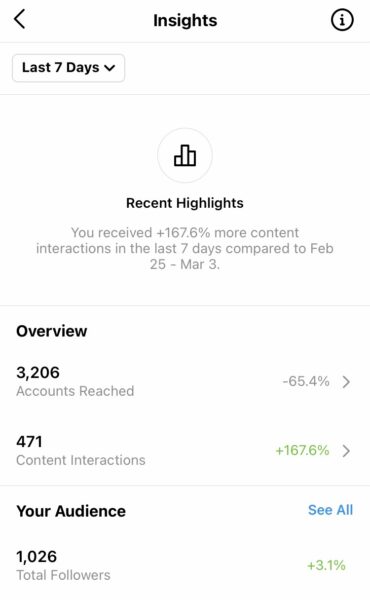A detailed screenshot of social media performance insights, likely from Instagram, displays comprehensive analytics regarding the page's recent activity. The top header features a familiar navigation layout with a back arrow in the top-left corner, a centered title "Insights" in bold black text, and an information button represented by a lowercase 'i' encircled in the top-right corner.

Beneath the header, a dropdown box labeled "Last 7 days" is positioned to the left, allowing users to select the time range for which they want to view insights. The main section of the screen is dominated by a "Recent Highlights" summary presented in monochrome. It indicates a significant 167.6% increase in content interactions over the last seven days compared to the previous week (February 25th to March 3rd).

The dashboard provides an overview of various performance metrics, including accounts reached, content interactions, audience demographics, and follower count, with each metric's current trend direction indicated.